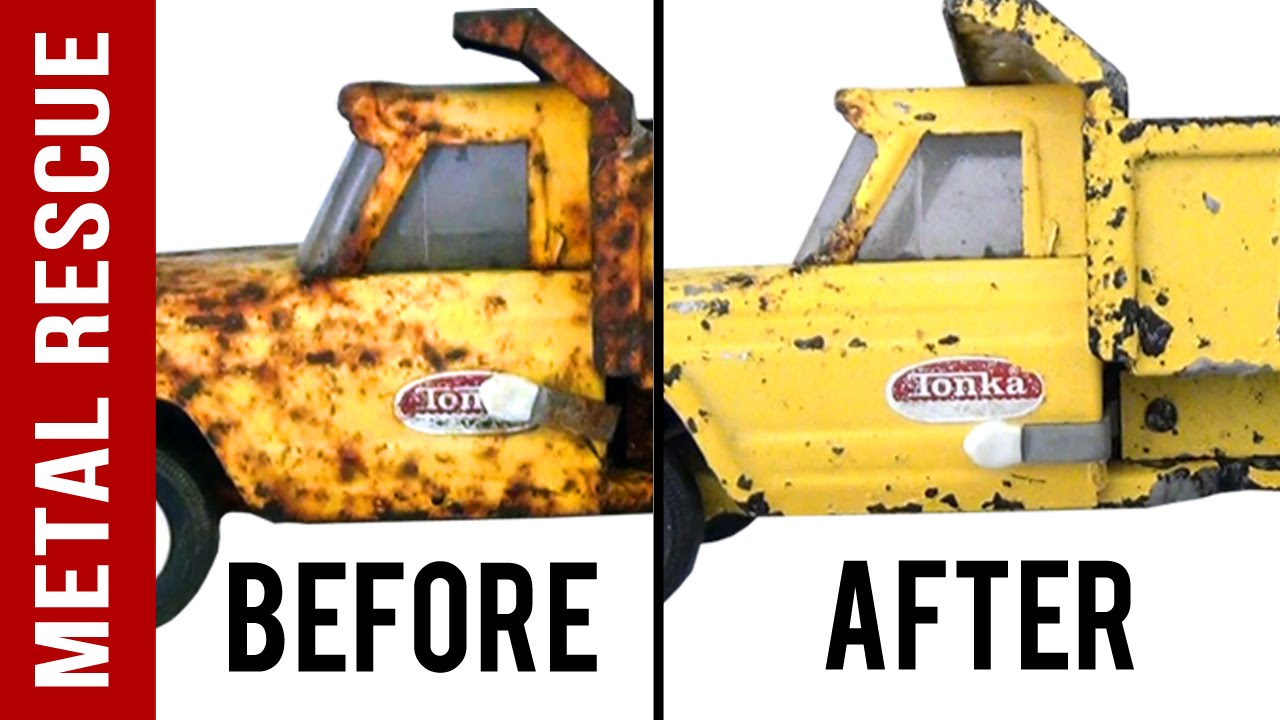The image is a rectangular advertisement measuring roughly six inches wide and three inches high, divided into left and right sections by a thin black vertical bar. On the left side, a vibrant red background features the bold, white text "METAL RESCUE." Below this, a "Before" image depicts the front half of an old metal Tonka dump truck. The truck's original yellow color is heavily marred by widespread brown rust spots, making it look battered and neglected, with its silver Tonka emblem partially obscured by corrosion.

To the right, an "After" image showcases the same Tonka truck after undergoing restoration. The truck's yellow paint appears much brighter, with most rust spots removed and only minor gray patches remaining. The once-rusted door handle is now fully cleaned and restored to its original silver color, clearly revealing the Tonka sticker in its entirety. Despite still showing signs of aging and play, the significant contrast between the "Before" and "After" images emphasizes the effectiveness of Metal Rescue's services.